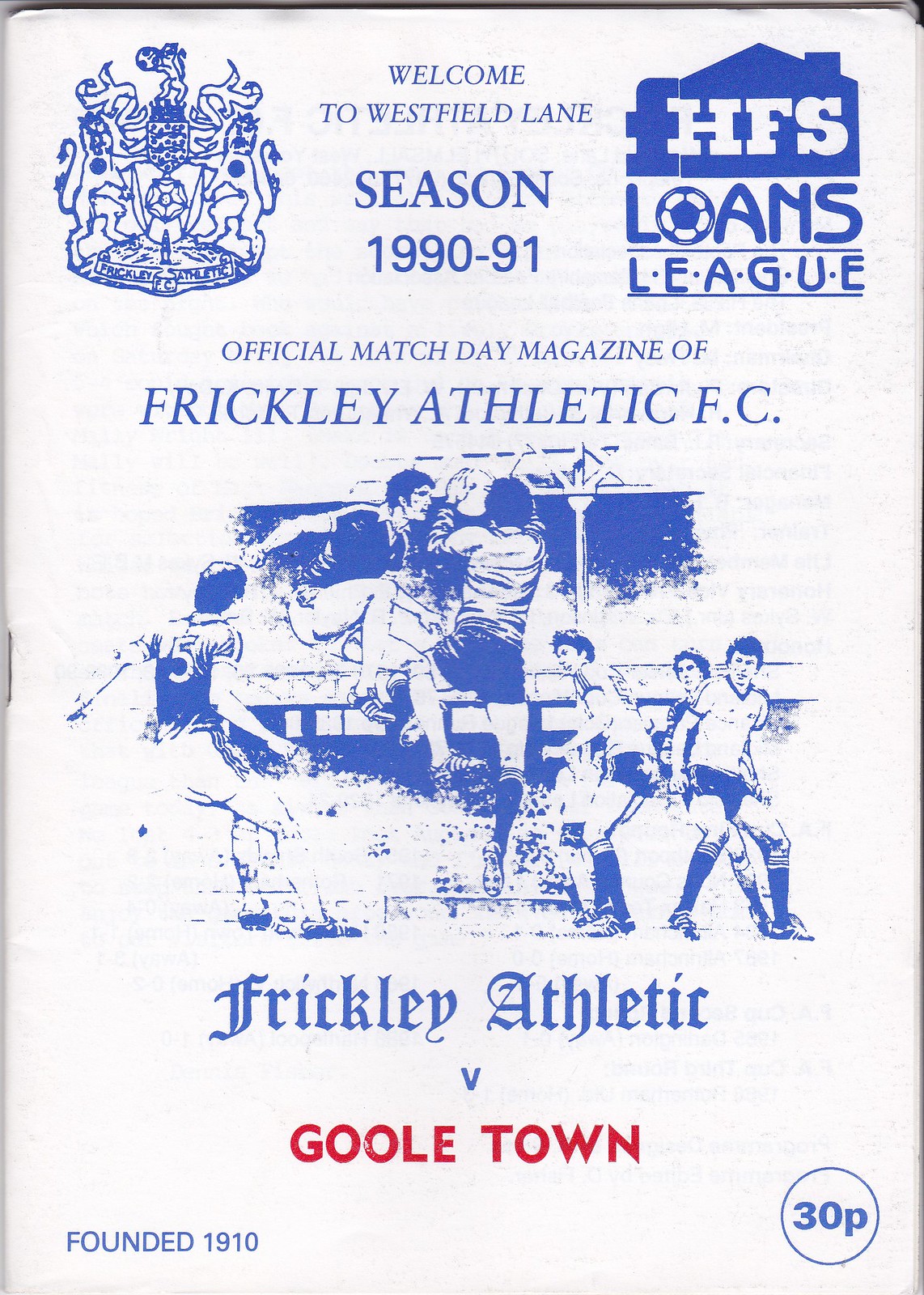The image is a blue and white flyer titled "Welcome to Westfield Lane, Season 1990-91," prominently displayed at the top. On the top left, there's an emblem featuring two white lions with crowns, flanking a blue shield with a cup in the center, and on the top right, there's a small blue house icon with the letters "HFS" inside. Below it, the text "Loans League" is written, with the "O" styled as a soccer ball. Directly underneath this section, the flyer identifies itself as the "Official Matchday Magazine of Frickley Athletic FC."

The central part of the flyer displays a black and white image of a soccer match between two teams, one in light-colored and the other in dark-colored uniforms. Specific details from the image include a player with the number five in white on their blue jersey. Below this photo, text in blue reads "Frickley Athletic vs." followed by "Goole Town" in red. In the bottom left corner, it states "Founded 1910," and in the bottom right corner, "30P" is written inside a blue circle. The overall theme of the flyer is dedicated to a soccer match, structured around the Frickley Athletic FC's activities.